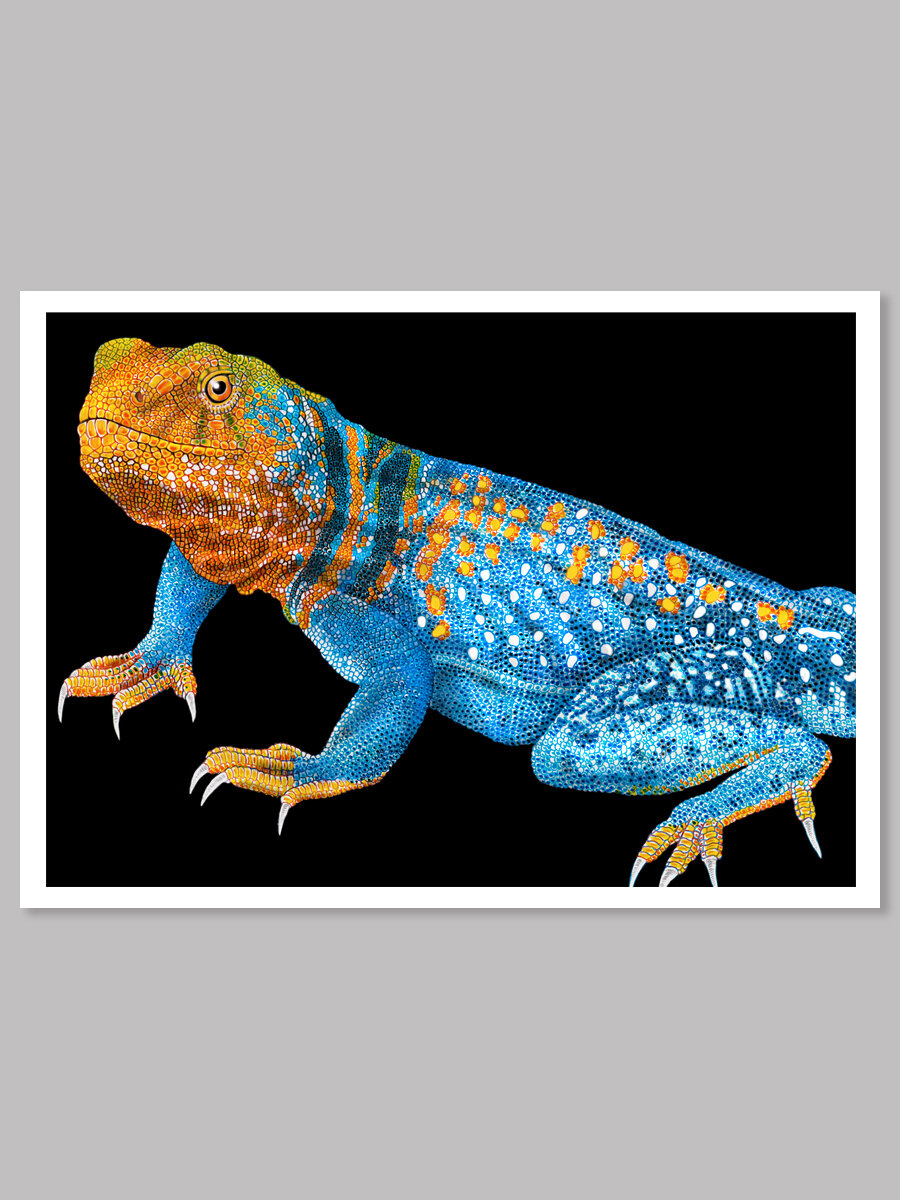The image features an iguana with a striking, multicolored appearance against a black background, framed by a white border on a gray canvas. The iguana's head is a vibrant mix of orange and green, with bright orange eyes. Its body, predominantly blue, is adorned with orange, yellow, and white spots. The iguana’s skin is scaly, with distinct white claws on its orange-tinted feet. Positioned in the center, the iguana is captured from the side, turning its head slightly towards the viewer, revealing its left eye and mouth. Only its two front legs and one hind leg are visible, as the image cuts off its tail and the rest of its body. The vivid details and absence of text emphasize the iguana’s unique and colorful features.